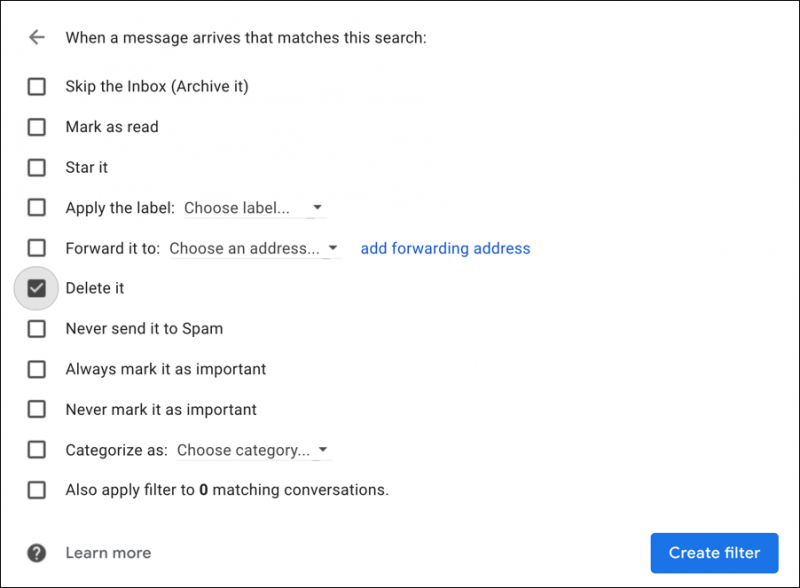The image depicts a detailed menu interface for creating a filter within Gmail. The white background suggests the interface is displayed in light mode. This menu allows users to set up automatic actions for incoming emails that match specific search criteria. Each action is preceded by a checkbox, indicating whether the action is selected or not.

Here are the actions listed, with the corresponding checkboxes:
- **Skip the Inbox (Archive it):** Unchecked
- **Mark as read:** Unchecked
- **Star it:** Unchecked
- **Apply the label:** Choose label (Unchecked)
- **Forward it to:** [Choose an address] (Unchecked, with an "Add forwarding address" link next to it)
- **Delete it:** Checked
- **Never send it to Spam:** Unchecked
- **Always mark it as important:** Unchecked
- **Never mark it as important:** Unchecked
- **Categorize as:** Choose category (Unchecked)
- **Also apply a filter to matching conversations:** Indicates "0 matching conversations" with the checkbox Unchecked

At the bottom of the menu, there is a "Learn more" link represented by a question mark inside a gray circle, and a prominent blue "Create filter" button in a rounded rectangle shape.

The consistent use of standard Google fonts and graphic elements strongly suggests this interface is part of Gmail, despite no explicit Google branding being present.